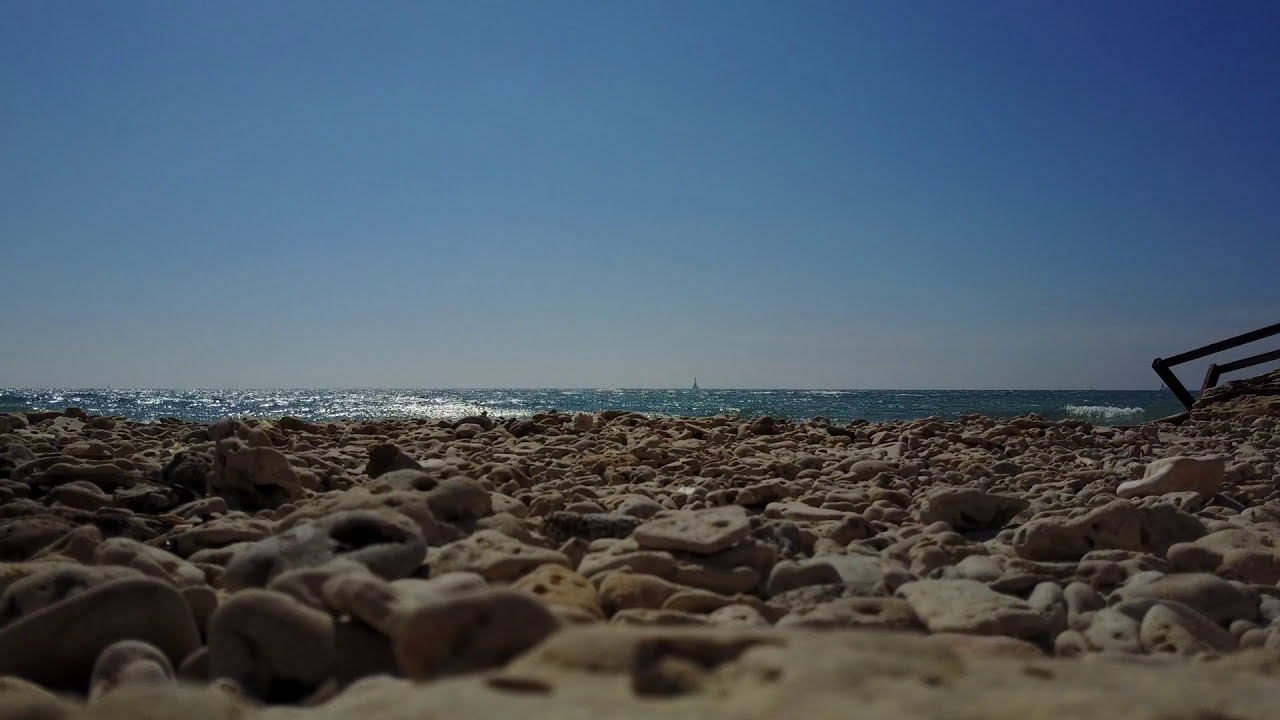In the foreground of this image, a rocky beach covered with various types of eroded rocks and shells stretches out. The rocks are a mix of mostly beige-gray and brown, some with multiple holes from erosion. These rocks come in different shapes, including square, round, and oval, and are scattered among the sand, which is natural and sandy-colored. Towards the right side, there is a wooden railing, possibly part of a walkway, leading down to this rocky shoreline. 

Beyond the rocks, a thin strip of deep, clear dark blue ocean is visible, with the sunlight reflecting off the surface and gentle waves rolling in. In the far distance, on the clear blue horizon, a large sailboat can be seen with its triangular sail faintly visible, or it could possibly be a building or a buoy. It is a sunny day with no visible sun but a clear blue sky. The image captures the intricate details of the rocks and shells up close, contrasting with the serene ocean and distant horizon.